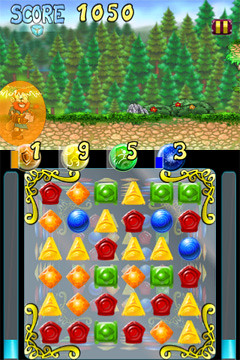The image depicts a vibrant and colorful screenshot from a video game akin to Bejeweled. At the center is a 6x6 grid filled with various brightly colored jewels, including yellow triangles, orange diamonds, ruby red hexagons, green squares, and blue circles, arranged for the player to match. Specifically, on top of the board are one orange, nine yellow, five green, and three blue jewels. Above the board, a score of 1,050 is prominently displayed in yellow, under the word "Score" written in blue. In the upper right corner, a small pause button comprised of two vertical yellow dashes on a purple square is visible. The backdrop features animated green trees and rocks, creating a natural ambiance. Additionally, there are blue progress bars on the left side indicating minor progress. The treasure chest icon, possibly for daily rewards, and the overall layout suggest an engaging and dynamic matching game.